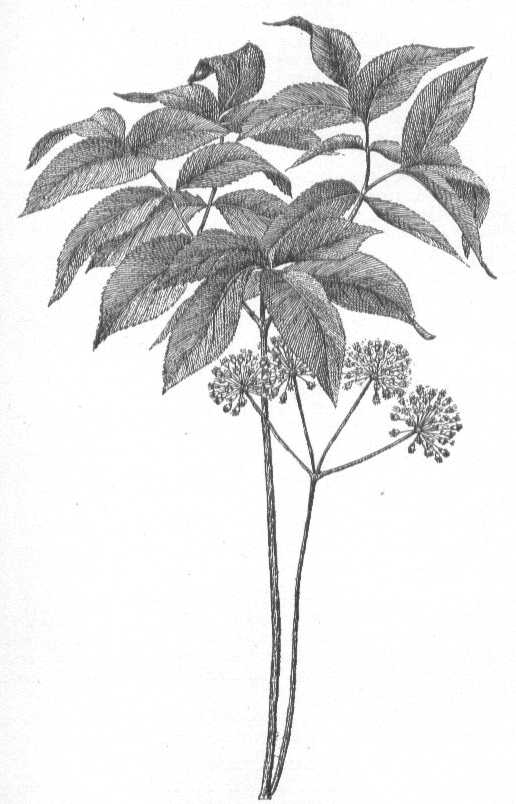The image is a detailed, black and white hand-drawn sketch of a single plant with two main stems. The shorter stem on the right rises up and branches into four smaller stems, each ending in a fluffy, dandelion-like flower. The larger stem on the left extends higher than the right and also branches off into several stems adorned with numerous leaves, varying in size and direction. The leaves and stems exhibit intricate shading to suggest depth and texture. The entire composition, seemingly created with pencil, sits against a white background, evoking an impression of an outdoor scene without any textual elements.